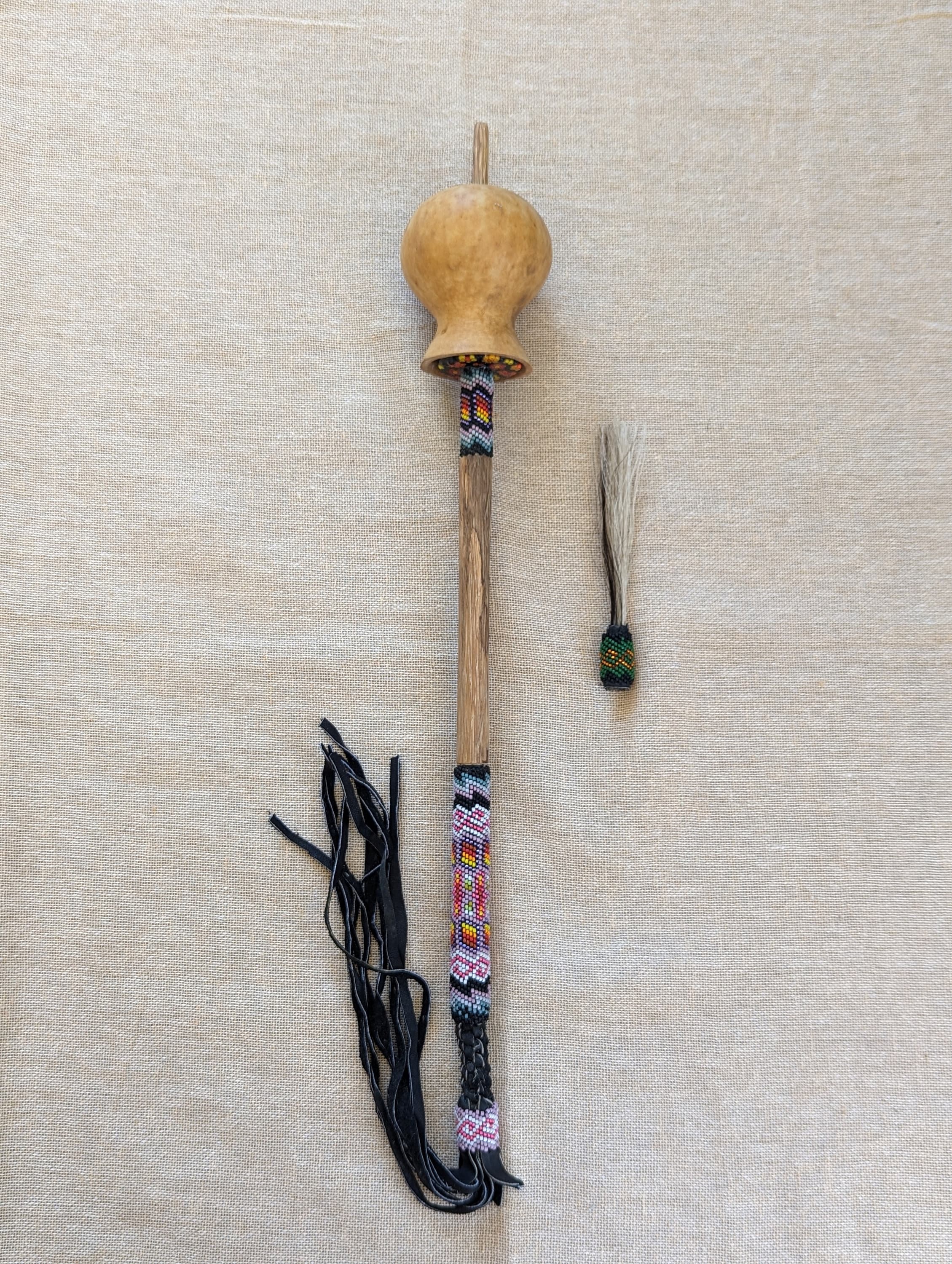The photograph features a finely crafted object resembling a Tibetan prayer wheel without the actual wheel, consisting of a wooden stick adorned with intricate, colorful patterns. These patterns are concentrated at the bottom of the stick and continue upwards towards a bulbous, doorknob-like structure on the top. The decorative handle has a vibrant native pattern with an array of colors including blues, reds, purples, yellows, pinks, and oranges. Attached to the bottom of the stick are numerous strands or tentacles made from string or leather. The object is set against a heavily grained white wooden surface or a piece of white paper mimicking a wood grain design. Right next to the primary object, there's a small, green, gold, and black bell-like item tied to a string, featuring what appears to be natural white and black animal hairs emerging from its top.